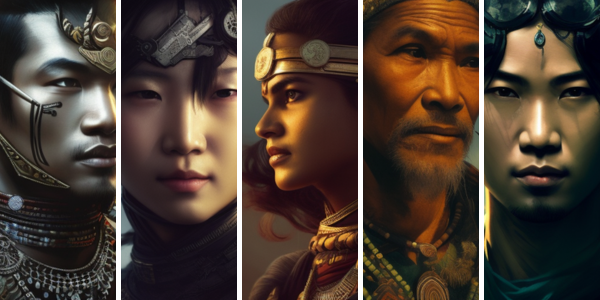This intricate image appears to be a form of digital art, possibly created using augmented reality (AR) technology or a sophisticated 3D modeling computer program, evoking a slight sense of the uncanny. The artwork seems to be influenced by Asian designs, with a strong inclination toward Filipino or Taiwanese aesthetic elements rather than Chinese. 

The scene depicts five individuals, each representing ancient, tribal folk heroes from a pre-industrial age, characterized by the use of traditional weapons such as bows, arrows, and spears. From left to right, the characters include a young man, a young woman, another young woman, an elderly man, and another young man. The detailed styling and cultural elements suggest a deep connection to historical craftsmanship and traditional narratives.